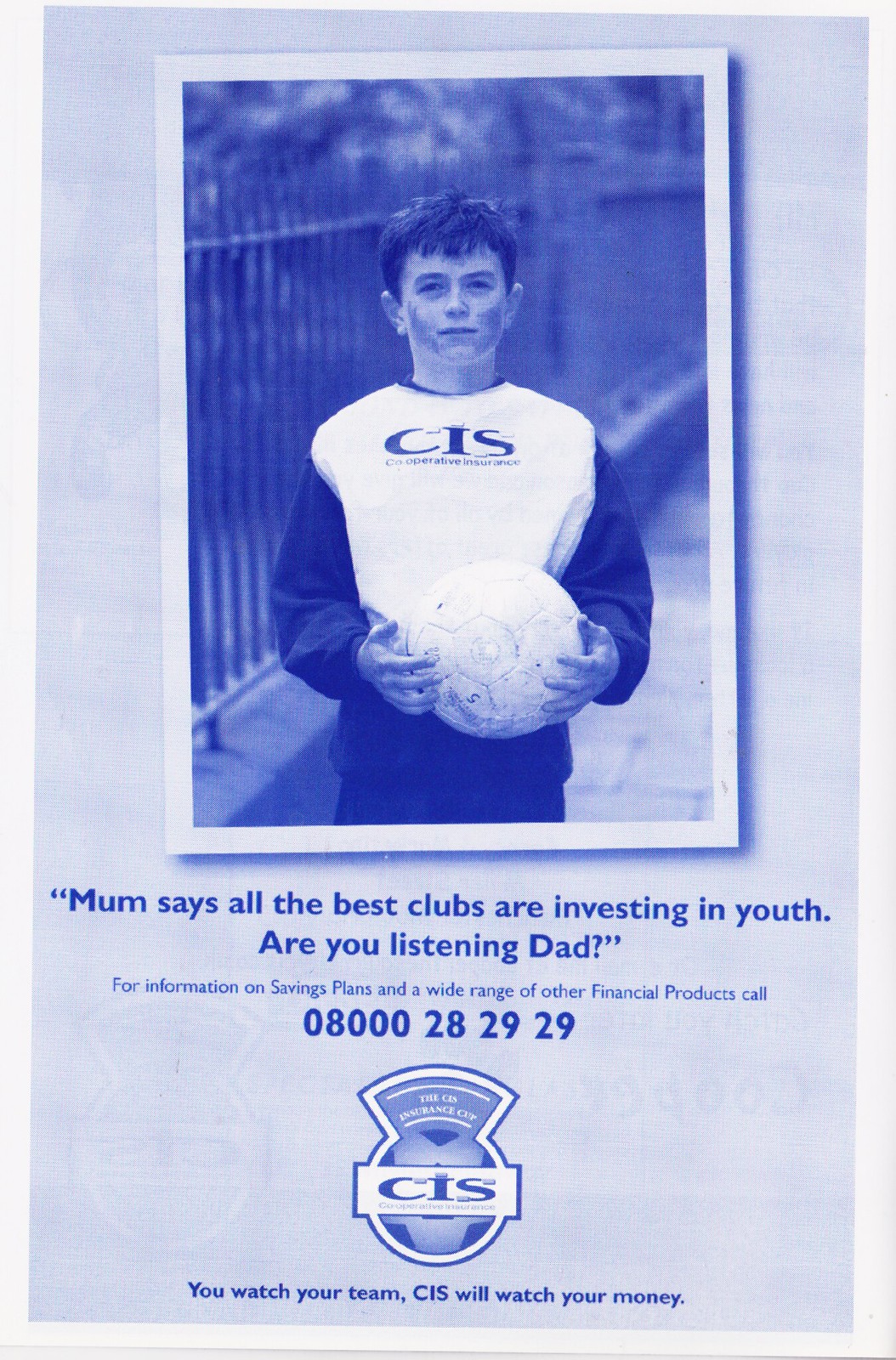The image is a scanned advertisement from a football or soccer magazine. Predominantly blue and white, it features a young boy holding a white soccer ball, staring directly at the camera. The child is dressed in a white jersey with "CIS" prominently printed in the center, paired with dark sleeves of a long-sleeved jacket and dark shorts or pants. He has marks on his cheeks, possibly for sun protection, and short hair. Behind him is a steel fence and concrete ground, suggesting an outdoor setting.

The primary text, positioned under the boy, reads in blue: "Mom says all the best clubs are investing in youth. Are you listening, Dad?" This is followed by smaller text providing information on savings plans and other financial products, alongside a phone number: 0800-28-2929. Near the bottom, there's a logo of a blue globe with a crown and a white banner across it that also reads "CIS." Beneath this, it states: "You watch your team, CIS will watch your money." The entire layout and text are rendered in shades of blue, with unprinted areas remaining white.